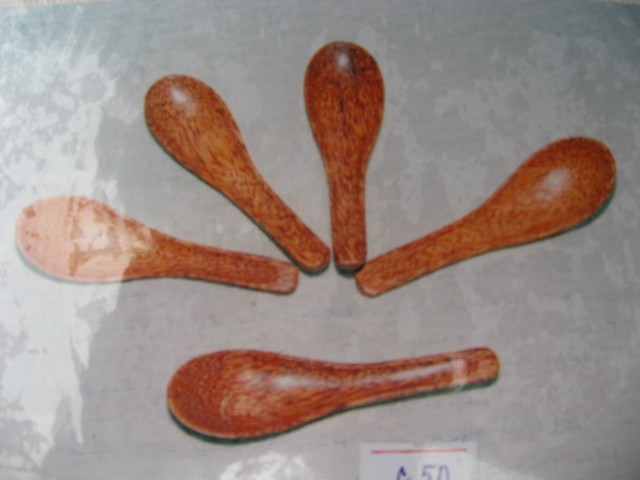This is a color photograph depicting five wooden spoons with short handles, likely of Asian design characterized by their wide, deep scoops. Each spoon beautifully showcases the wood grain, with a dark brown hue accented by touches of yellow. The spoons are arranged in a fan-like pattern: four centrally positioned, fanning out from left to right, with a fifth spoon laid horizontally beneath them, its bowl facing left. The image quality is notably poor, suggesting it could be an older photograph. The spoons appear to be displayed under a reflective glass or plastic cover, as indicated by a reflective area on the far left. At the bottom of the photograph, slightly right of center, there is a partial price tag visible, showing the number "50" and an unidentifiable symbol. No people are present in the image.